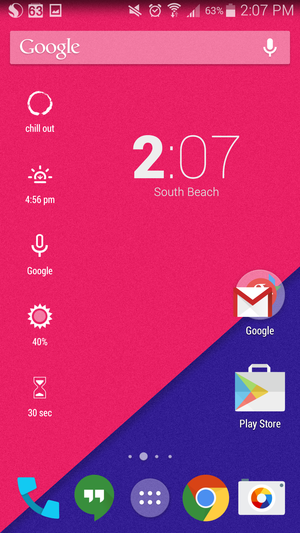In this image, we see a series of screenshots featuring a smartphone's interface. On the status bar at the top of the screen, several icons are clearly visible: a mute icon indicating the phone is on silent mode, a calendar icon, a Snapdragon processor icon, a WiFi signal icon showing full signal strength, a network signal icon with 3 out of 5 bars, a battery level indicator displaying 63%, and the current time, which reads 2:07 PM. 

The screen also features various texts including "chill out," "4:56 PM," "Google," "40% humidity," and a timer set to 10 seconds. Several app icons are prominently displayed, including Google Chrome, Play Store, Gmail, Phone app, Hangouts, and the Camera app. The details in the screenshot provide a snapshot of the device's status and activities at a specific moment.